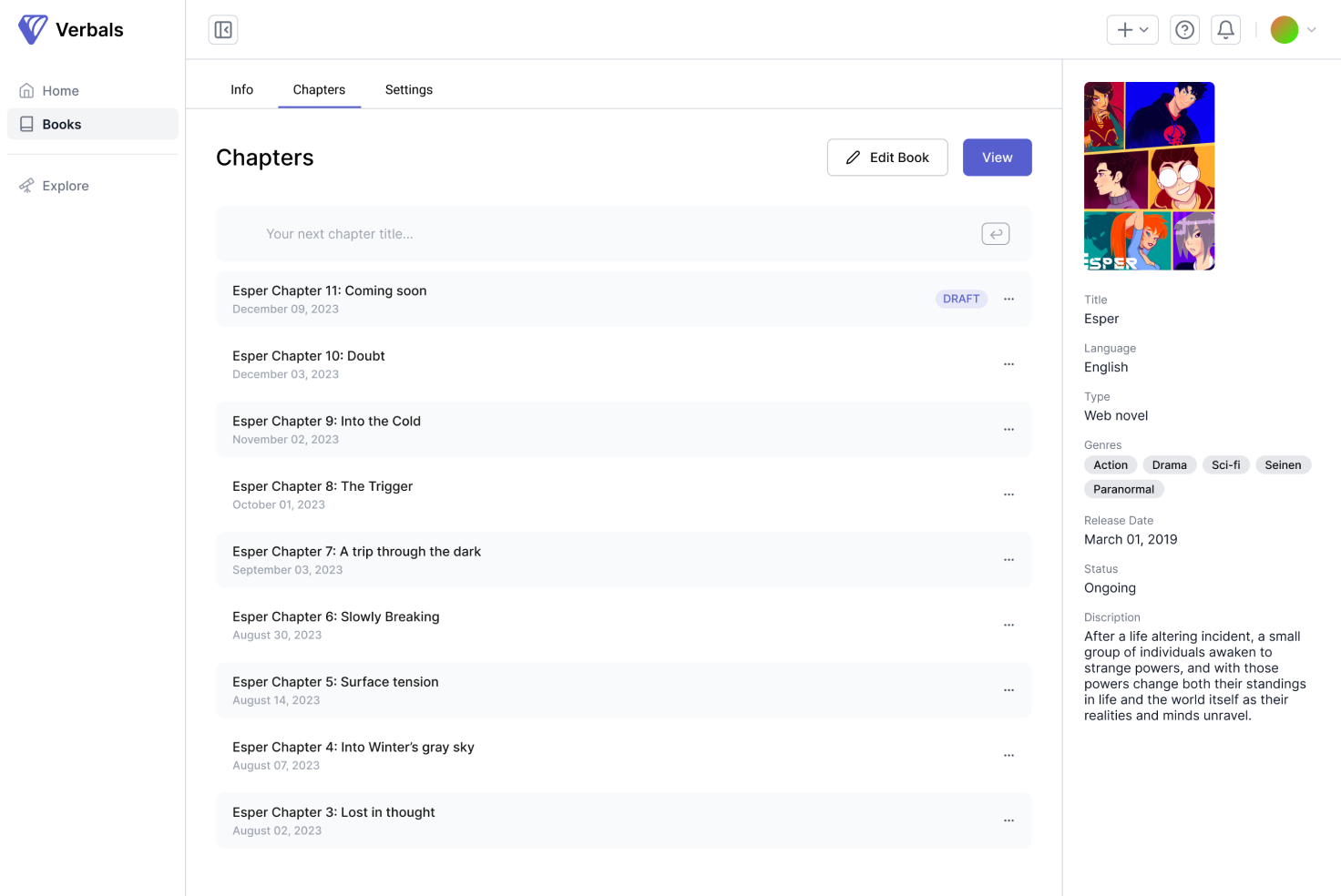This is a webpage from Verbalos, depicted in meticulous detail. In the upper left-hand corner, we find the word "Verbalos" in black, accompanied by their icon to the left, which features a purple and white design. Spanning across the top of the screen, there are three categories available: Info, Chapters, and Settings. "Chapters" has been selected; it is underlined in purple, highlighting its active status.

The content is organized in alternating white and light blue banners. The word "Chapters" is displayed in black text on a white background, accompanied by an "Edit the Book" button and a blue "View" button to the right. Beneath this, a light blue banner delivers the prompt "Your Next Chapter Title..." in black text.

Following this, the page continues with a series of chapters listed on alternating blue and white banners. The first light blue banner reads "Chapter 11: Coming Soon" in black text, featuring a "Draft" button on the far right. Underneath, a white banner lists "Chapter 10: Doubt." The next light blue banner shows "Chapter 9: Into the Cold," followed by "Chapter 8: The Trigger" on a white background. This alternating color pattern persists, with "Chapter 7: A Trip Through the Dark" on a light blue banner, continuing down through chapter 3.

This detailed layout showcases an organized and visually engaging way to navigate through the contents of a book-in-progress on Verbalos.